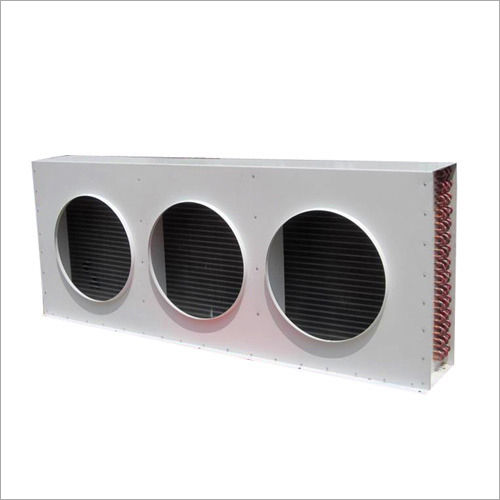This image showcases a rectangular, orthogonal-view HVAC or air conditioning equipment, possibly a radiator. The structure is made of white metal and features three large circular cut-outs along its left side, precisely aligned vertically. The circles are set against a backdrop of gray horizontal lines. Along the right edge of the device, a complex network of copper tubes and connectors is visible, looping and running the length of the box. Numerous screws are lined up along the edges and between the circles. The piece is designed for heating or cooling purposes, incorporating copper coils within its metal frame. The entire assembly is presented against a plain white background.